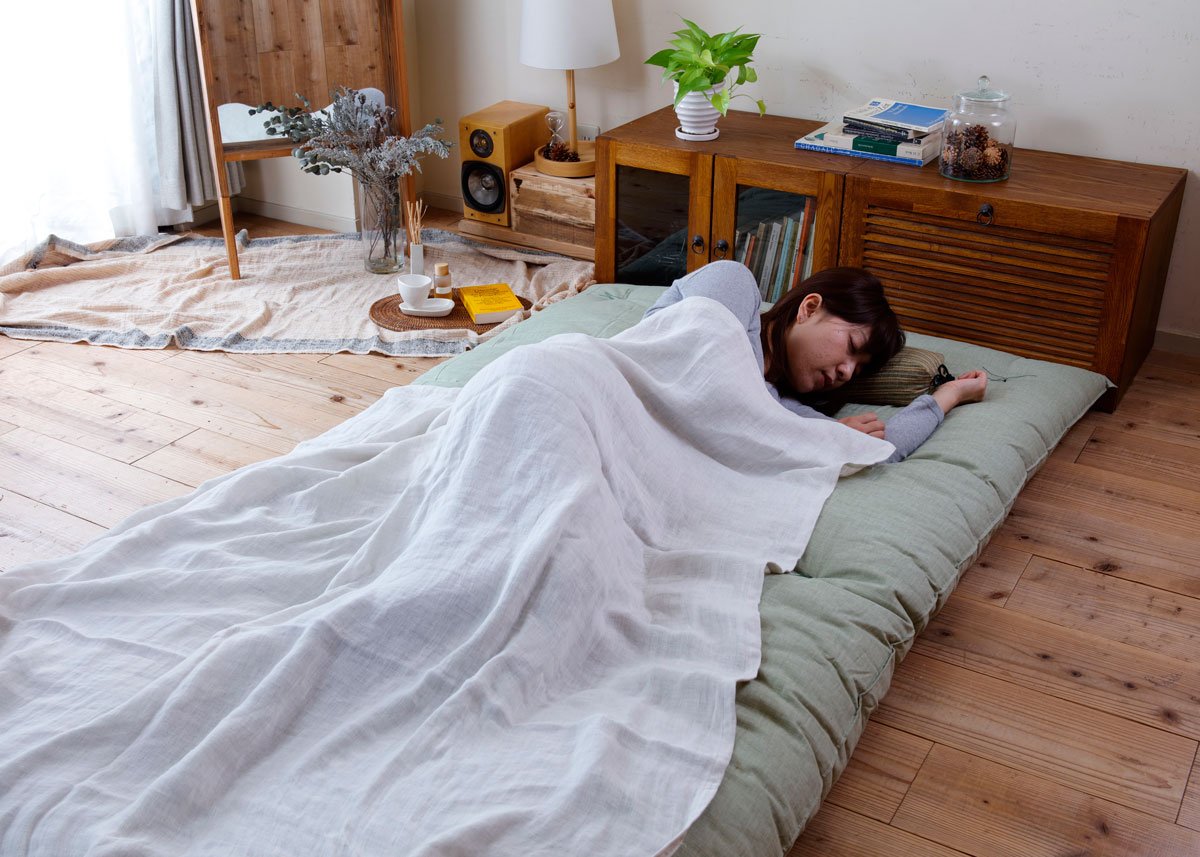The photograph captures a serene bedroom scene featuring an Asian woman sleeping peacefully on a sage green mattress pad, directly on a light wooden floor. She is covered with a white linen sheet and wears a light blue long-sleeved shirt, lying on her left side with her head resting on a small rolled pillow. In the background, a brown wooden cabinet with three doors—two of which are glass-paneled, revealing books inside—anchors the left side of the image. Atop this cabinet sits a white pot containing a plant, several books, and a decorative jar with dried flowers. Positioned near the cabinet is a small white lamp and a speaker. In the back left corner of the room, there's a towel or tablecloth laid on the floor with an oval tray holding a book, a mug with a saucer, and another vase containing blue dried flowers and sticks. The cabinet appears to have a drawer that opens outwards, providing additional storage. The overall atmosphere suggests a cozy and well-organized living space, blending elements of both a bedroom and a living room.